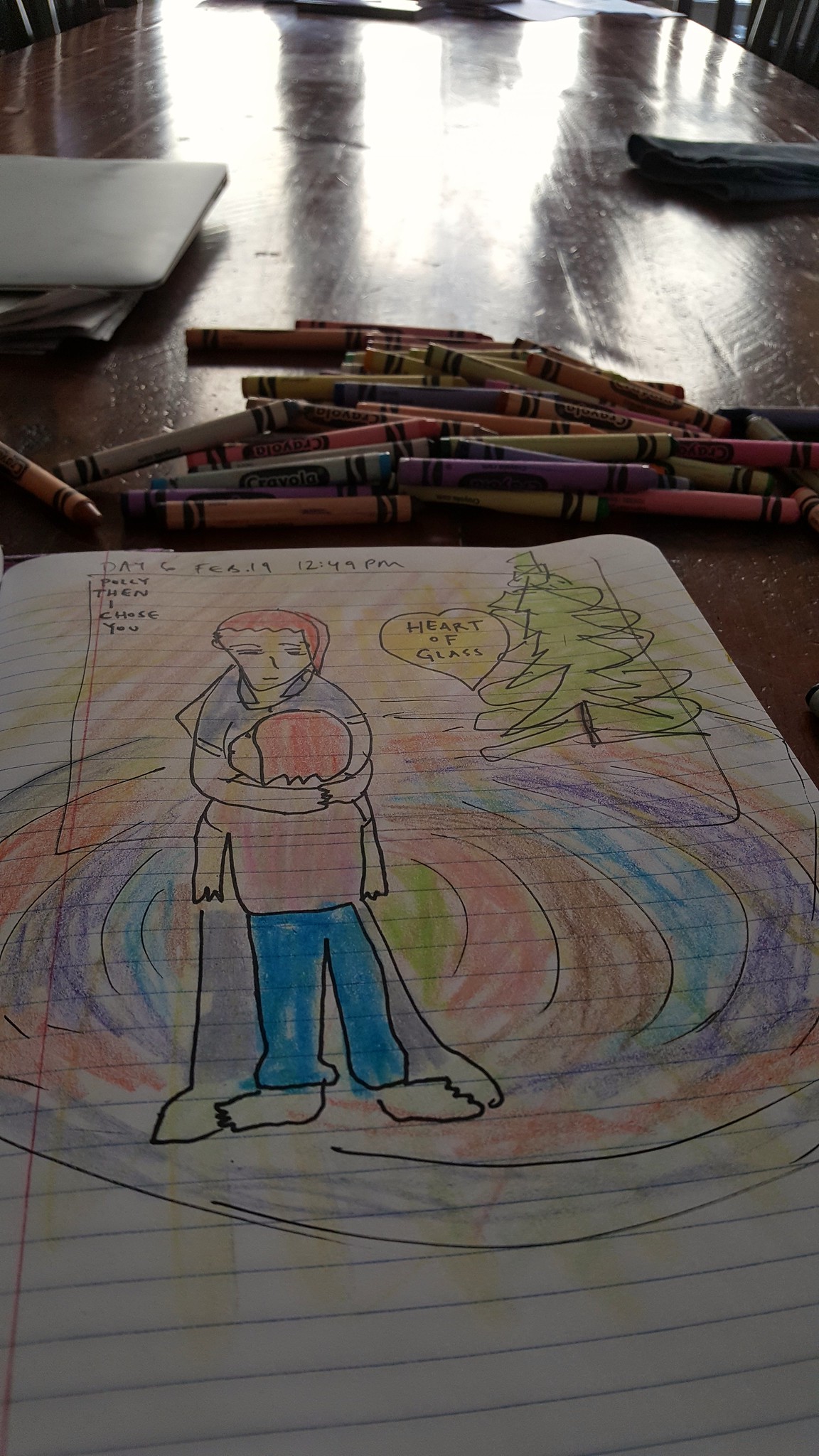A highly detailed drawing on white, blue-lined notebook paper, featuring a red line running vertically along the left margin, is set against a glossy, brown wooden table. In the background, a closed gray laptop is visible. A pile of crayons in a spectrum of colors, reminiscent of a rainbow, lies nearby on the table. The central image on the notebook paper depicts a woman with red hair embracing a child, who also has red hair. The woman is dressed in a blue shirt and pants, while the child wears a pink shirt and blue pants. Below them, a vibrant, rainbow-colored swirl adds a dynamic element to the composition. To the right, a green pine tree is positioned beside a yellow heart inscribed with the words "Heart of Glass." In the upper left corner of the page, the text "Day 6, February 19th, 12:49 PM. Polly, then I choose you." is written, adding a temporal and personal element to the artwork.